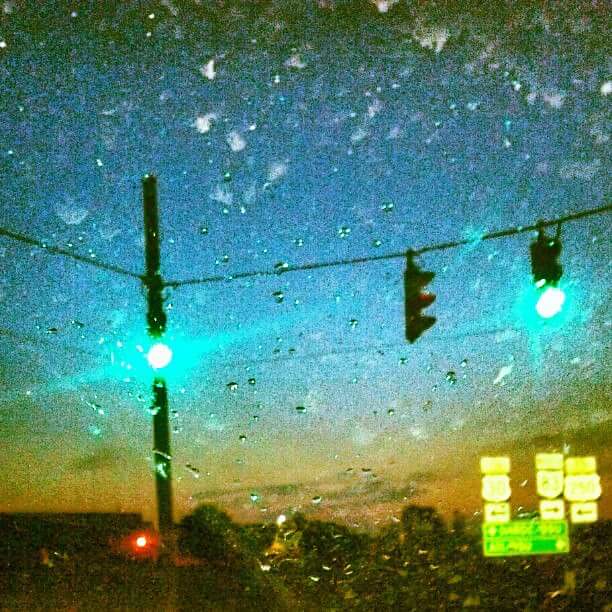The photograph is a square image, seemingly taken from inside a car through a rain-streaked window. The scene outside is a post-sunset cityscape, captured during or just after a rain. The window is covered in reflective, clear raindrops, giving the image a hazy, slightly blurred quality. In the sky, dark gray clouds hover against a beautiful gradient of deep blue fading into yellow, orange, and red as the sun has recently set. A dark black cable stretches across the scene, supporting traffic lights that show a bright green light on both the left and right sides, with the center light facing away but likely illuminated red. In the distance, another red light glows near some indistinct buildings. Various highway signs, though small and unclear, suggest directions with arrows pointing left and right, and one green sign with white text. A dark pole holds up one of the traffic lights, emphasizing the urban setting amidst the moody, rain-drenched atmosphere.